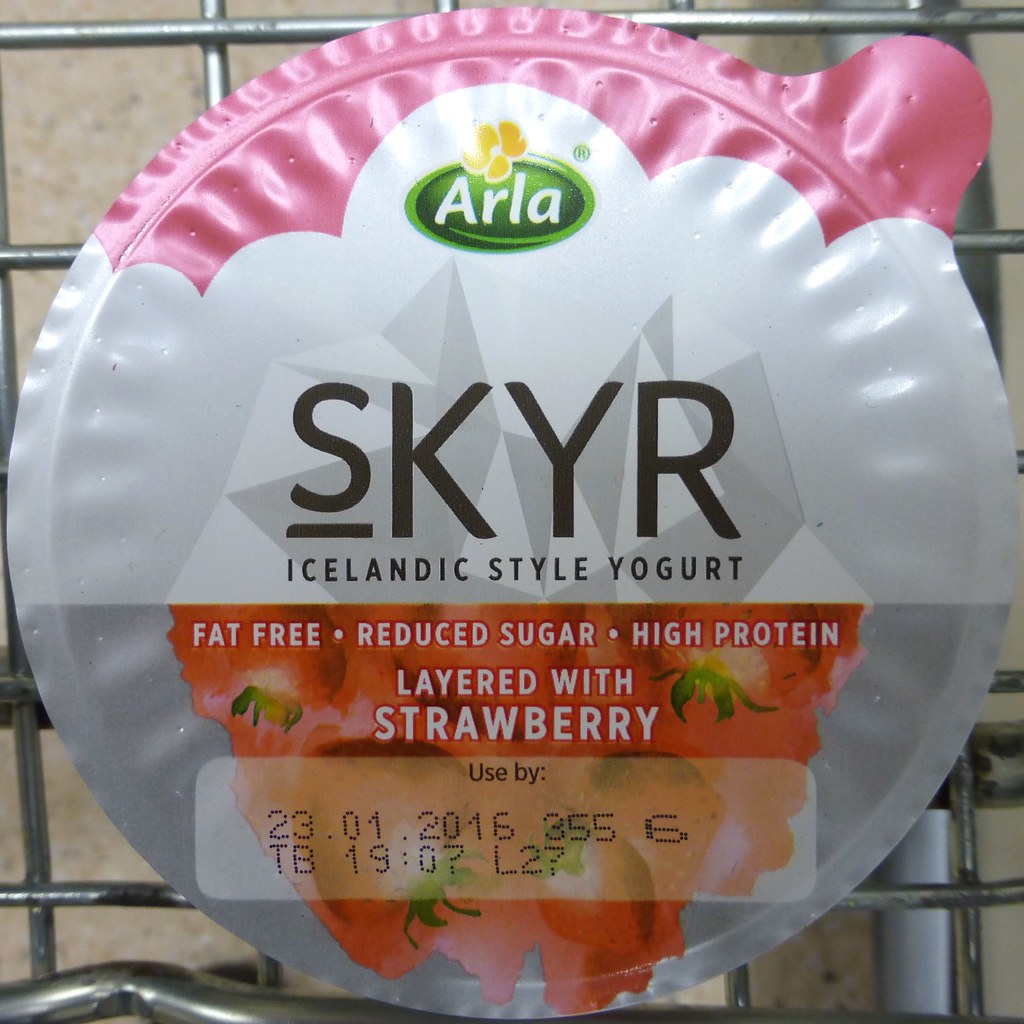This image is a detailed close-up of the top of a yogurt cup, specifically an Icelandic style yogurt from the brand Arla. The cup is predominantly white with a narrow pink border along the top. A pull tab for opening the yogurt, also pink, is located in the upper right corner. The brand name "Arla" is prominently displayed in white font within a green oval in the top middle area, adorned with a yellow petaled flower.

Dominating the center in large black letters is the word "SKYR." Just below, smaller text reads "Icelandic style yogurt." A horizontal line separates this from the lower section, where the background turns gray and features an image of strawberries. Superimposed on the fruit are the descriptors "fat-free, reduced sugar, high protein" in white text. Further down, it states "layered with strawberry." At the very bottom, there's a "Use By" strip displaying a date of January 23rd, 2016, along with additional characters and a timestamp reading "19:07 L 27."

The yogurt cup appears to be positioned on a metal rack, possibly the inside of a shopping cart or a dish rack, suggesting the image was taken in a store or grocery environment.